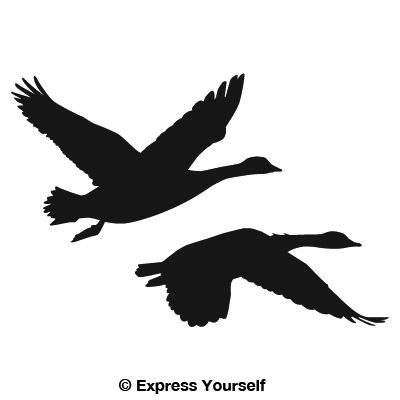This black and white image features a detailed silhouette of two geese in flight against a blank white background. The geese are depicted entirely in black and are oriented towards the right side of the image. The lead goose, positioned lower, has its wings in a downward stroke, with individual feathers visible along the edges. The rear goose is slightly above, with its wings in an upward V-shape, indicating an upward stroke. Although the fine details of their faces are not visible due to the silhouettes, the realistic representation of their wings and tails offers insight into their form and motion. This striking contrast is complemented by the black text "Express Yourself" with a copyright symbol at the very bottom of the image.